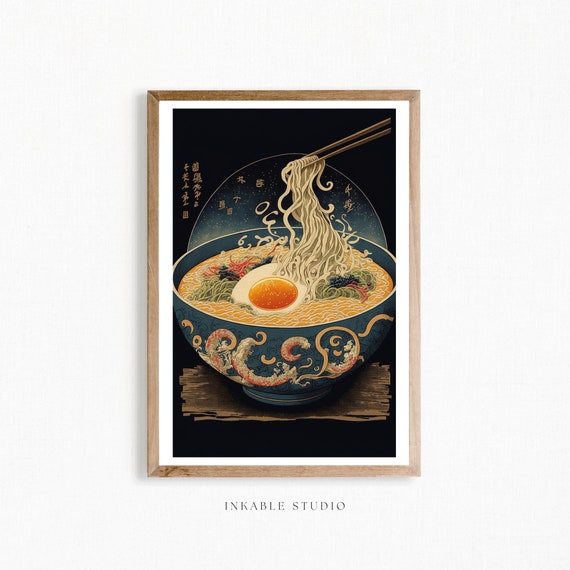This framed illustration by Inkable Studio depicts an ornate bowl of ramen against a black background. The image features a pair of chopsticks lifting a bundle of noodles from the amber-colored broth within the bowl. The artistic bowl, adorned with shrimp-like shapes and octopus tentacles, also contains a poached egg and various garnishes, including greens and possible fish eggs. The ramen sits on a brown surface that appears to be smeared with seaweed or cloth. Behind the bowl, there is an arch of sparkly elements and Japanese lettering, adding to the Asian aesthetic of the piece. The artwork is framed with a wooden exterior border and a white interior border, and the text "Inkable Studio" appears below the illustration.